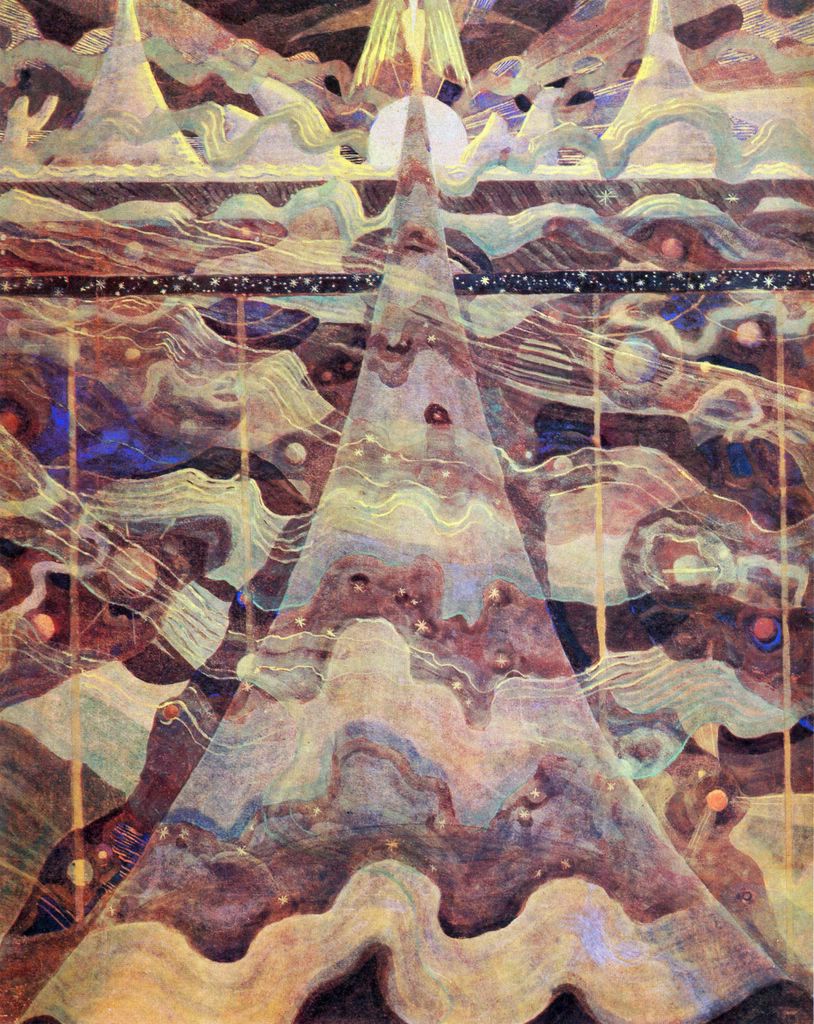This captivating painting showcases a surreal, fantastical scene that merges elements of a mystical forest and an ethereal landscape. Dominated by a large, tree-like shape that resembles a Christmas tree, the composition is incredibly detailed with layers of wavy, cloth-like textures creating a sense of depth. The tree, adorned with Christmas balls, stands majestically in the center, its triangular form extending from the bottom corners upward. At the pinnacle of the tree-like structure is an angel with golden wings, arms at its sides, set against a luminous three-fourths white moon. The color scheme is remarkably unique, with hues of blue, beige, yellow, light green, and red blending harmoniously throughout. Surrounding the central figure, the scene is filled with other uniquely shaped trees and mountain peaks that fade into a dark, surrealistic background. Adding to the fantasy element, a large, footbridge-like path ascends into the sky, arching over the glowing moon and mingling with beams of yellow light and starry ripples. This intricate and imaginative painting beautifully combines forest and celestial themes into a singular, mesmerizing landscape.